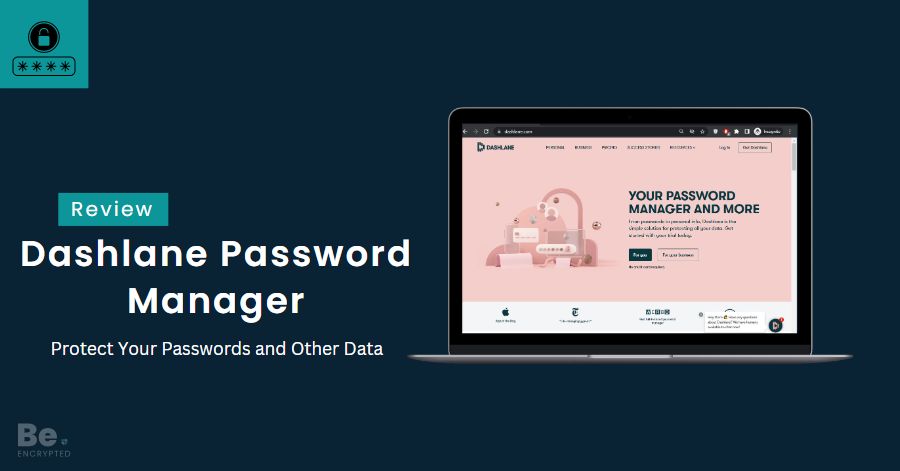In this image, the background is a deep dark blue, creating a contrasting backdrop for the elements in the foreground. On the left side, there is a lighter blue box featuring an icon of a lock accompanied by four stars, which signifies security and reliability. Adjacent to this box, towards the right, is a laptop displaying a website.

The website's primary color scheme is pink. On the left side of the laptop screen, there's a blue box with a review label. Beneath this label, the text reads "Dashlane password manager - protect your passwords and other data." Towards the bottom left corner of the screen, the phrase "Be encrypted" is visible, emphasizing security features.

Displayed prominently on the laptop screen, the website text states "Dashlane - your password manager and more," indicating the page's main focus. The website appears to be viewed in a standard Chrome browser window, which is in incognito mode as indicated by typical visual cues. 

Various other elements are present on the webpage, including different categories and a login button. Additionally, there are notable logos such as an Apple logo and a 'Times' logo towards the bottom, lending credibility. In the bottom right corner, there is a chat bot text, suggesting available customer support or interactive help features.